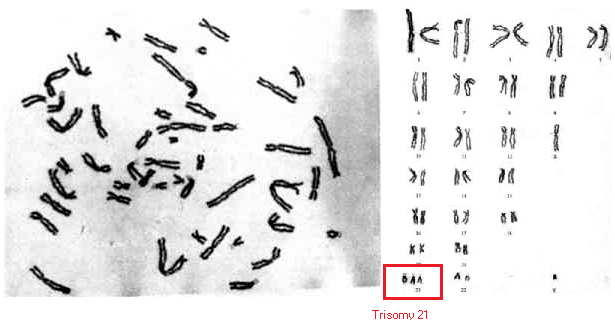This image, seemingly from a textbook or educational material, is divided into two sections to form a complete rectangle with a clear scientific theme. The left section features a microscopic image in black and white, depicting around 20 small organisms resembling thick, segmented worms or chromosomes, intricately interweaving and crossing over each other. On the right section, set against a plain white background, is a detailed chart showcasing various types of chromosomes, each uniquely shaped and labeled with minuscule font. A specific chromosome, identified as "Trisomy 21," is outlined distinctly in a red rectangular box at the bottom of the chart, drawing the viewer's attention to this anomaly. The precise labeling and structured formatting of the chart, paired with the detailed microscopic imagery, underscore the educational and scientific nature of the illustration.